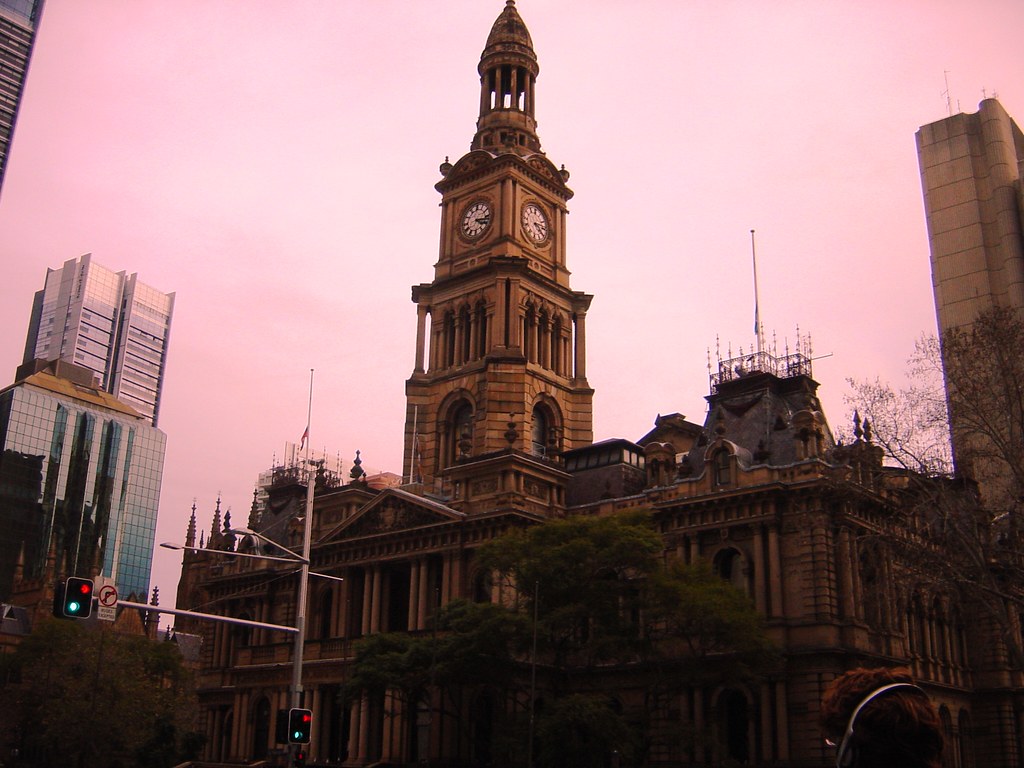The image showcases a cityscape captured at dusk, with a captivating pink-orange sky hinting at sunset. Dominating the scene is a grand Victorian-style building made of brown bricks, featuring a prominent clock tower with intricate architecture, adorned with cornices and rounded archways. The clock tower, reminiscent of Big Ben in its grandeur, extends into the skyline, topped by a dome, with the clock hands showing a few minutes past three. To the left of this historical structure stands a towering modern skyscraper with numerous mirror-like glass windows that reflect the evening light. On the right, contrasting sharply with both buildings, is a stark, cement slab structure with an austere, 1980s architectural style. A stoplight in the foreground displays both green and red lights, and a "no right turn" sign is visible. At the base of the clock tower, a traveler with red hair and headphones looks up, seemingly admiring the majestic old tower juxtaposed against the modern office buildings.